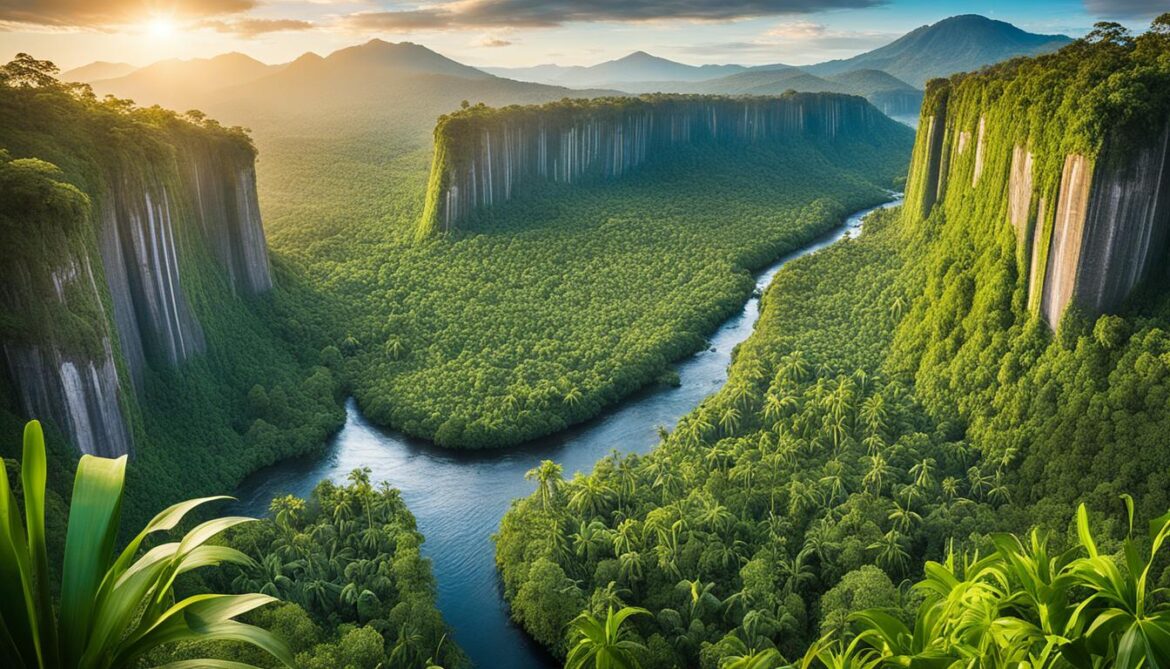The horizontally aligned rectangular computer-generated image showcases a partly cloudy sky with the sun shining in the upper left. The sky features a blend of gray and white clouds with pockets of blue visible. Below the sky, a distant outline of mountains can be seen. In the middle of the image, a tall rock wall or vertical cliff, adorned with green vegetation, stands prominently. Surrounding the rock wall, dense green bushes and trees cover the scenery. A narrow stream of water cuts through this verdant landscape, widening slightly in the lower left area before splitting into two directions: one stream continues downward, while the other veers toward the lower left side. The right side prominently features tree tops, with another rock formation topped with green vegetation. Large palm leaves are notable in the lower left corner of the image, adding to the lushness of the scene. The overall view is a rich, natural landscape with no human presence.